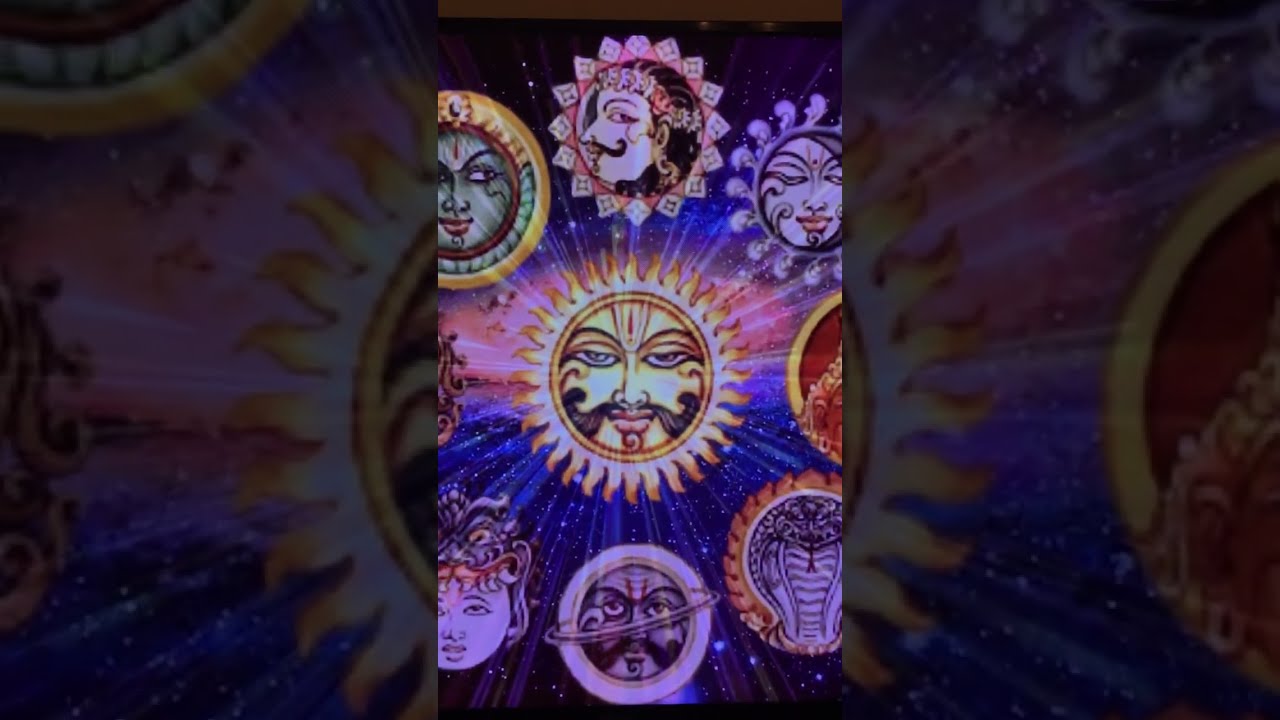In this image, a vibrant and mystical design captures the eye, centralizing around a radiant Sun bearing a human face complete with a mustache. The Sun, rendered in yellow, red, orange, and white hues, is strategically positioned in the very center of the frame. Encircling the Sun are six distinct icons, resembling what could be the hours on a clock. Among these icons are different faces and a cobra, each enclosed within small circles. The background evokes a cosmic atmosphere with shades of blue, purple, white, black, and salmon, enhancing the ethereal aesthetic of the image. The overall design appears to draw on Eastern spiritual symbolism, presenting a captivating blend of colors and motifs in a seemingly digital format. There is no text within the image, and it seems to have been captured from a mobile device, suggesting it was shared online.